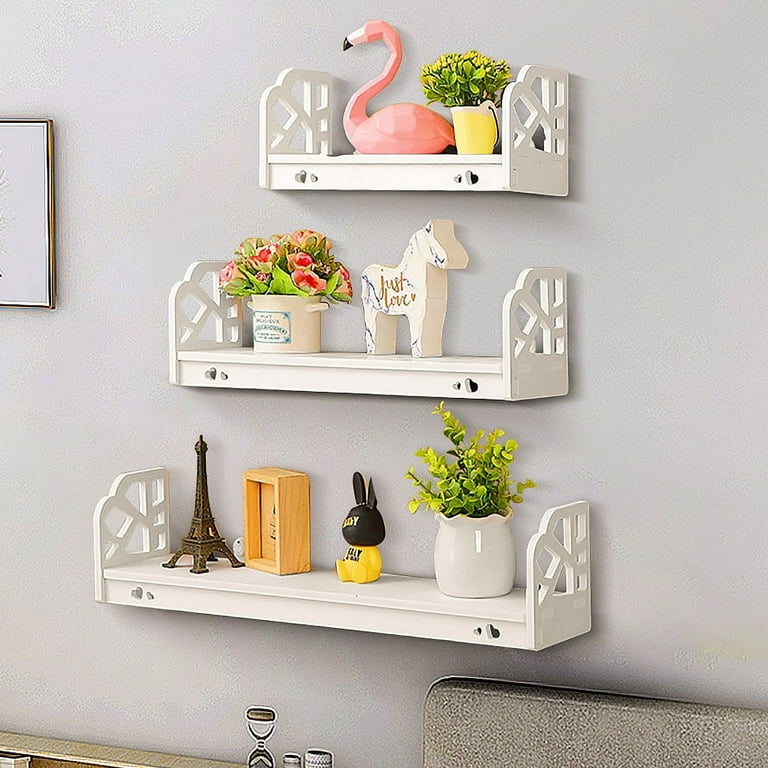The image depicts a wall adorned with three white shelves, each progressively shorter in length from bottom to top. The bottom shelf spans the widest, followed by a medium-sized middle shelf, and the top shelf is the narrowest. The top shelf features a pink wooden flamingo with a white beak tipped in black. Beside the flamingo, a small yellow bucket-like vase holds a green plant. The middle shelf hosts a carved white horse with the words "Just Love" written in gold along its side, accompanied by a white pot containing red, pink, and green flowers. The bottom shelf displays a white vase with green leaves, a yellow-bodied figurine resembling a rabbit with a black head and tall pointy ears, a brown wooden box, and a miniature metal Eiffel Tower. The image has a unique effect that gives it a somewhat computer-generated appearance, and the camera angle reveals a small portion of a mirror or framed art piece on the wall's left edge. Additional objects, including a small hourglass and cylindrical bottles, can be seen resting on a small wooden shelf at the bottom left corner of the image.